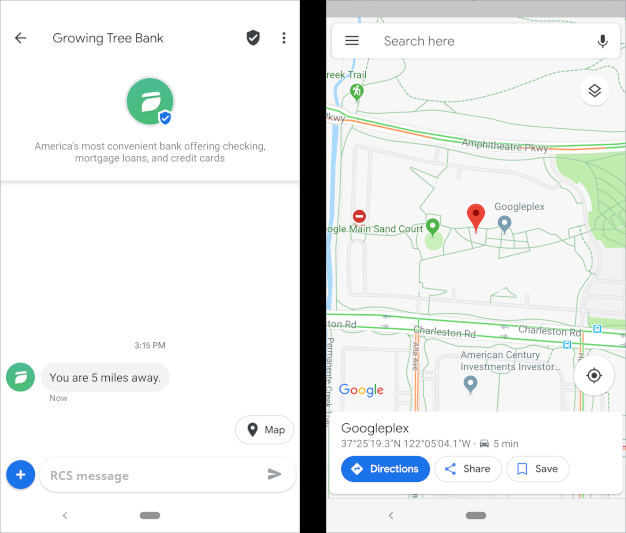The image depicts the interface of a banking website for "Growing Tree Bank." On the left side of the screen, there is a black circular icon with a checkmark inside, accompanied by three dots. An arrow indicates navigational options to go left. Within the green circle, a smaller blue circle with a checkmark represents a leaf, aligning with the bank's nature-themed branding. Text on the image proclaims "America's Most Convenient Bank Offering Checking, Mortgage Loans, and Credit Cards." Below, additional text notes the time "3:15 PM" and the information "you are five miles away." A map pin and the label "RCS Message" with a blue plus sign can also be seen.

On the right side of the interface, there is a detailed map showing the location of "Growing Tree Bank," marked with a red pin. At the top, a search bar includes an option to enable voice input. Below the search bar, three horizontal lines provide additional search functionalities. The map outlines various streets and is powered by Google, with the Google logo displayed underneath. Options for "Plaques," "Directions," "Share," and "Save" are available in circular icons at the bottom of the map.